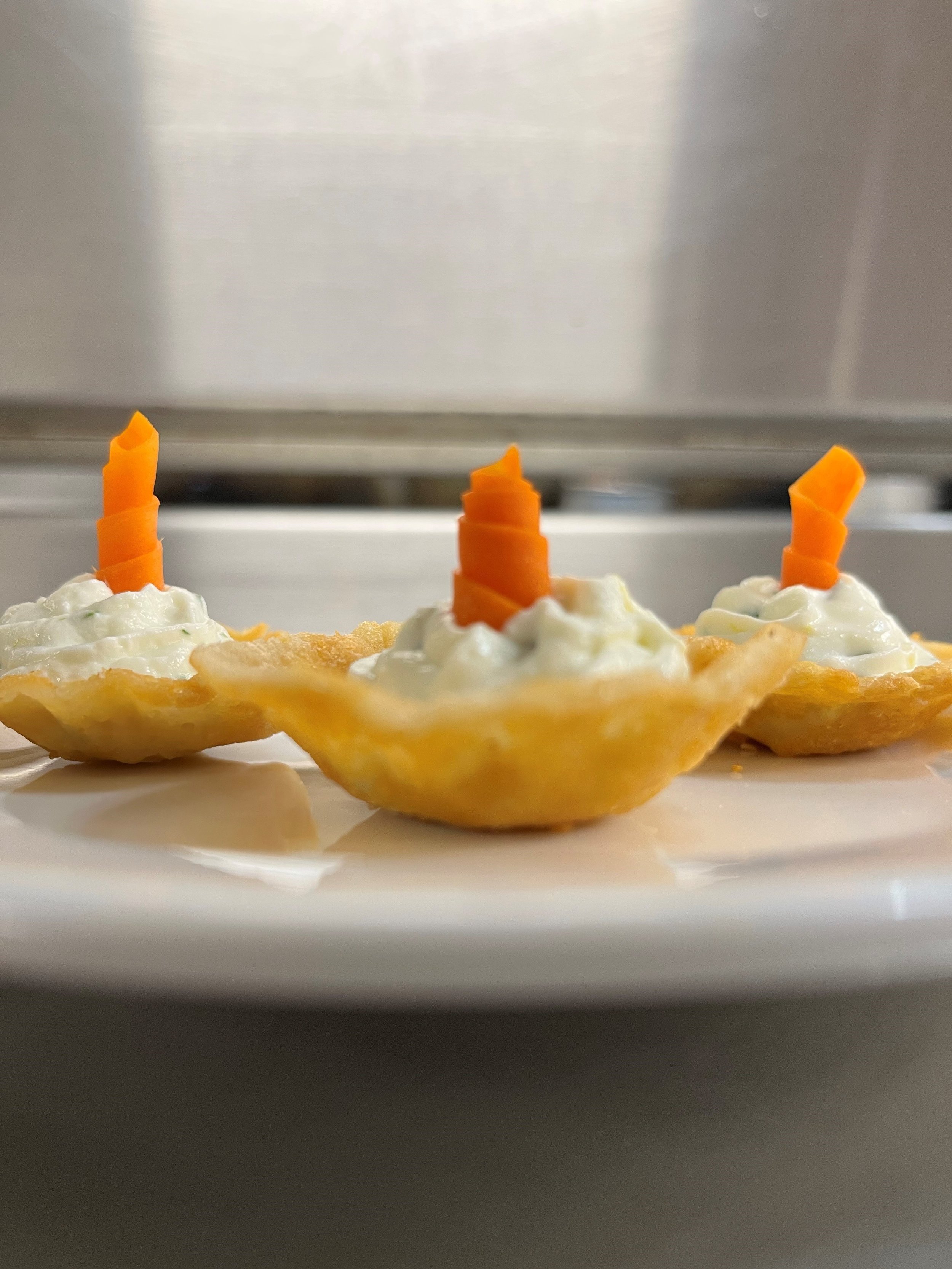This image features a close-up of three unique appetizers displayed on a white plate. Each appetizer consists of a small, round pastry shell at the bottom, filled with a creamy white substance that resembles mayonnaise or cream cheese. Intricately placed in the center of each is a spiraled, peeled carrot, creating a visual that resembles an orange rind twist. The background is slightly out of focus, giving a glimpse of a possible stainless steel or metallic surface, adding to the presentation's sleek aesthetic. These miniature creations bear a resemblance to tiny cakes or hors d'oeuvres, captivating the eye with their elegant and inviting appearance.